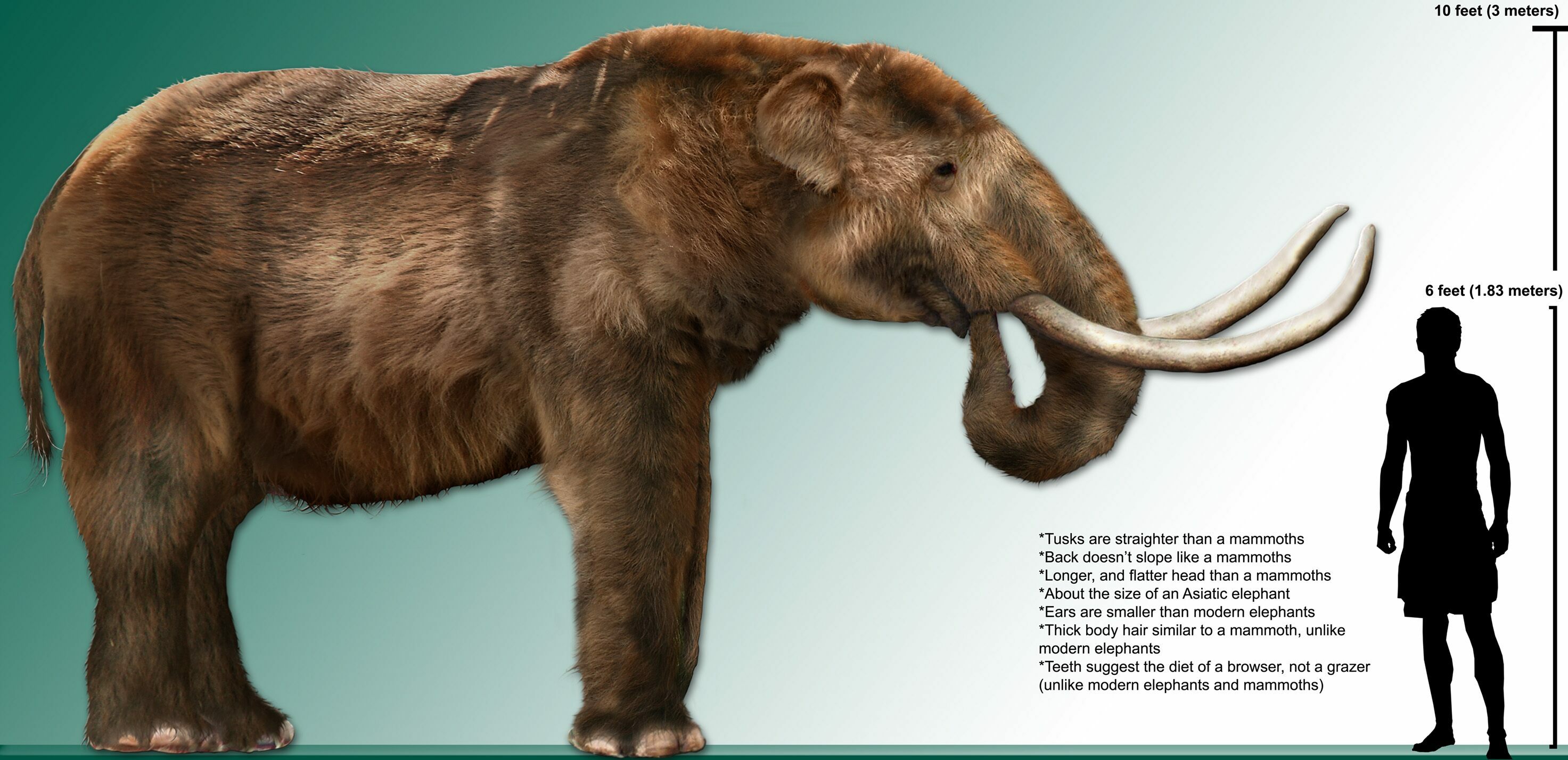The picture depicts a detailed comparative illustration with a distinctly colored background transitioning from dark teal on the left to white on the right. On the left side stands a realistic, fuzzy, brown-furred woolly mammoth, while on the right, there's a silhouette of a person. Above the individual's head, the text indicates a height of "6 feet, 1.83 meters," and at the top of the mammoth's back, it states "10 feet, 3 meters." Between the mammoth and the person, textual annotations describe various features of the animal: straighter tusks than a typical mammoth, a back that doesn't slope, a longer and flatter head, ears smaller than those of modern elephants, and thick body hair akin to that of a mammoth but unlike modern elephants. It also notes that the teeth suggest a browsing diet, different from the grazing habits of both modern elephants and mammoths. The animal is described as being about the size of an Asiatic elephant. This comparison highlights significant distinctions from both mammoths and modern elephants.